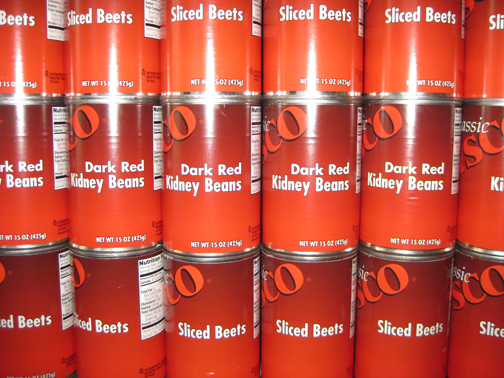The photograph showcases a vibrant and neatly arranged display of canned goods, consisting of three rows and six columns, totaling 18 cans. The cans are uniform in size, likely 15 ounces each, and feature a consistent, eye-catching color scheme—predominantly red with variations from a darker red at the top to a lighter red at the bottom. The top and bottom rows are labeled "Sliced Beets" in white lettering centered on an orange backdrop, while the middle row is designated "Dark Red Kidney Beans," also in white lettering. The manufacturer’s name on the cans is partially visible, ending with "SCO," and while some labels mention "classic," not all cans are positioned to fully display this detail. Additionally, the nutritional information is partially discernible on the right side of some cans, further enhancing the organizational detail of the display.